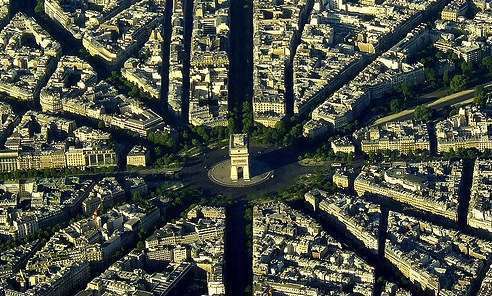This is an aerial view of the Place Charles de Gaulle in France, showcasing a sprawling traffic junction radiating from the iconic Arc de Triomphe at its center. The image captures the distinctive circular layout of the plaza, with several roads emanating outwards like spokes on a bicycle wheel, creating a web of connectivity across the city. The monument itself, a prominent white structure, stands majestically in the middle of the circular pad, surrounded by green trees. The surrounding roads vary in width, with the central ones being larger and busier, and as they spread out, they narrow down. The roads are connected by several narrow alleys or streets. The buildings adjacent to these roads appear mostly gray or light brown, blending with the urban landscape. On the left-hand side of the image, a noticeable row of large buildings is visible, likely commercial or prominent structures, while the other areas comprise primarily of residential buildings. The entire scene is presented without any text or borders, focusing purely on the intricate infrastructure and layout of this famous Parisian landmark.